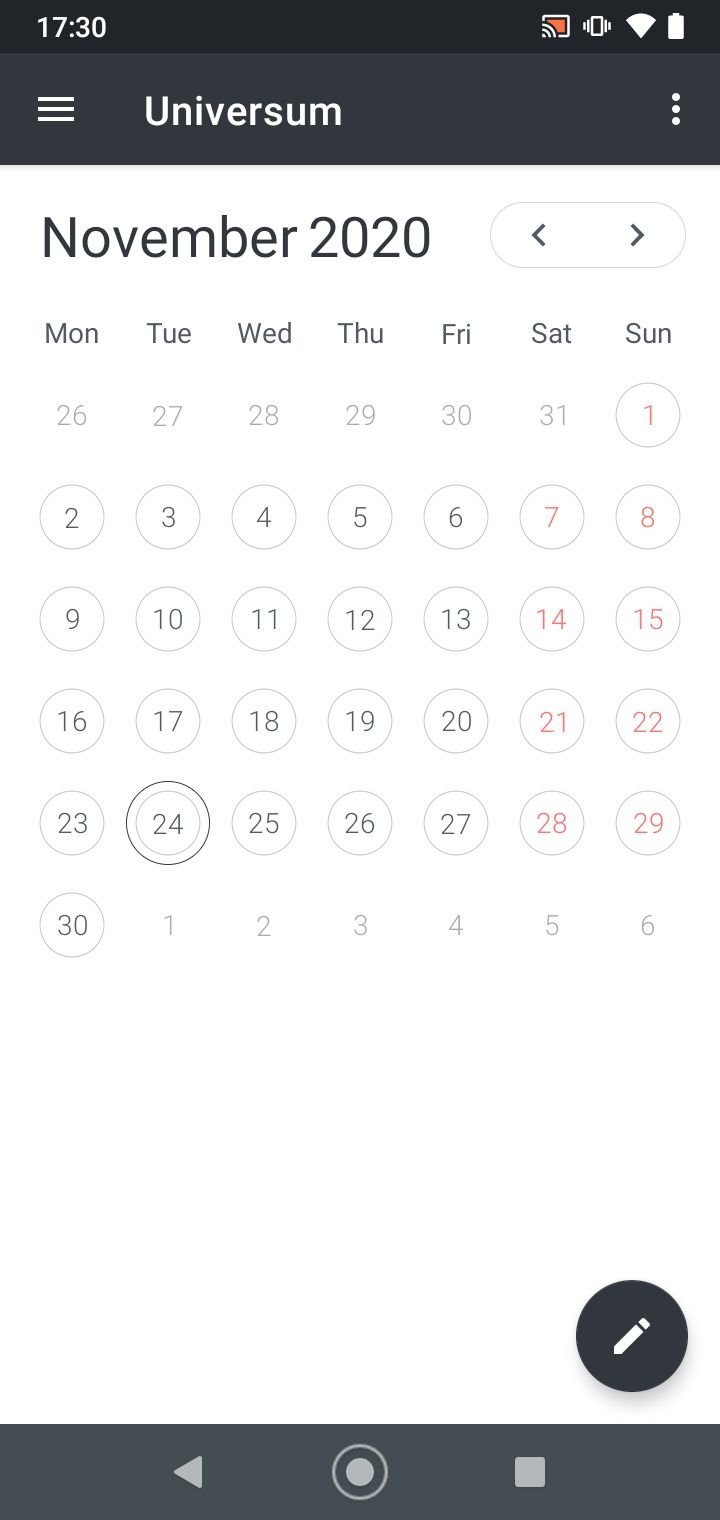The image is a screen capture of a calendar app displayed on a smartphone, taken at 17:30 as indicated in the top left corner. To the right of the time display are various status icons, including Wi-Fi signal bars, battery level, and a vibrate mode indicator, with additional function buttons aligned at the very top right of the screen.

At the center of the interface, "Universum" is prominently displayed in white text on a dark gray background. Just below this label is the header "November 2020," which introduces a monthly calendar view. The calendar is organized by weeks, with days of the week labeled from Monday through Sunday, running left to right. Each day in the month of November is represented by a black number within individual bubbles that span from 1 to 30. Any days from the preceding or following months are grayed out, creating a clear distinction.

The calendar's background is white, with weekdays marked in black numerals and weekends (Saturdays and Sundays) highlighted in red. 

Situated in the bottom right corner of the screen is a circular "create or edit" button, illustrated with a pencil icon. Directly below this button are navigation controls, including options to go back, return to the home screen, and a square button likely functioning as a pause or stop button.